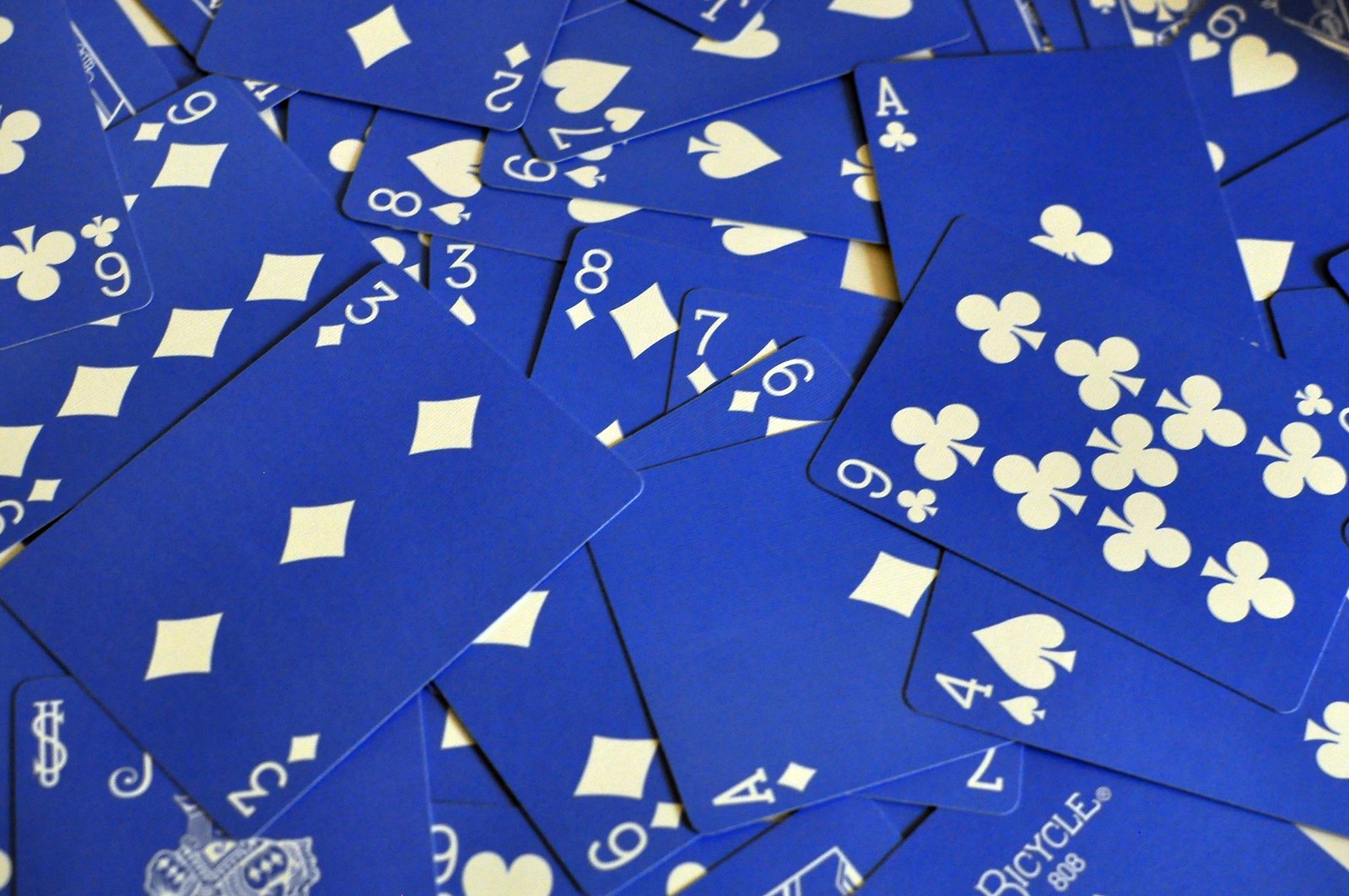This photograph showcases a distinctive set of Bicycle playing cards. Every card in the deck features a striking solid cobalt blue background. Contrasting sharply against this deep hue, the suits and letters are brilliantly white. The cards, all face-up, form an elaborate pile that fills the entire frame of the image. Among the visible cards on top are a 3 of Diamonds, a 9 of Clubs, a 4 of Spades, an Ace of Diamonds, an Ace of Spades, a 2 of Diamonds, a 7 of Hearts, another 9 of Clubs, a 3 of Spades, an 8 of Diamonds, an 8 of Hearts, a 6 of Diamonds, a 9 of Hearts, and a 6 of Hearts. The lighting, which casts a cool-toned illumination, emanates from the bottom right corner at a 45-degree angle, adding a crisp clarity and a subtle shadow effect to the scene. The meticulous arrangement and the unique color scheme of the cards make for a visually captivating display.